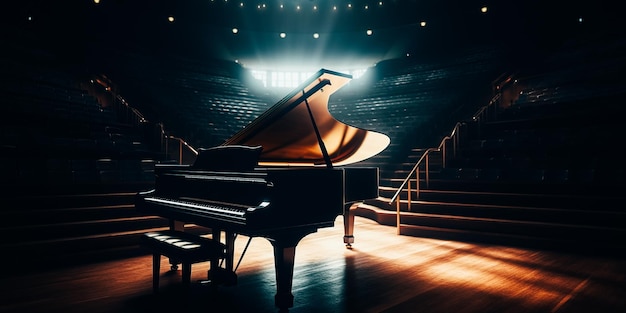The image depicts a grand piano centrally positioned on an elevated stage. Surrounding it is an expansive, empty audience area with tiered seating visible behind the piano. The stage is flanked by two staircases that ascend diagonally toward the upper right and left corners of the frame. Overhead, high windows filter daylight into the space, while stage lights hang from a darkened ceiling, casting dramatic shadows. The wooden floor beneath the piano gleams subtly, reflecting ambient light and enhancing the piano's finish. While the piano appears to be a dark shade, the interplay of light and shadow makes it difficult to discern whether it is black or brown. The overall scene is one of contrast, elegance, and serenity, showcasing the piano as the focal point amidst the harmonious blend of architectural elements and lighting.